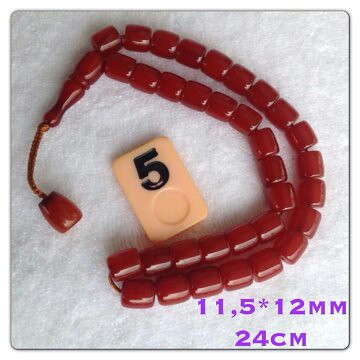The image captures a single strand of dark red, tube-like plastic beads strung on a thin, bronze-colored nylon cord. The beads are bluntly cut at both ends, giving them a slightly squared-off appearance. The strand is arranged in a loop, resembling a smile, with an additional bead hanging separately from the end. The background is white and appears to be cotton-like in texture. A small rectangular plastic card, in a tan-yellowy-orangey color, is placed next to the beads. The card features a black number 5 with a circle under it and lists the dimensions "11.5 x 12 millimeters, 24 centimeters" in purple text in the bottom right corner.